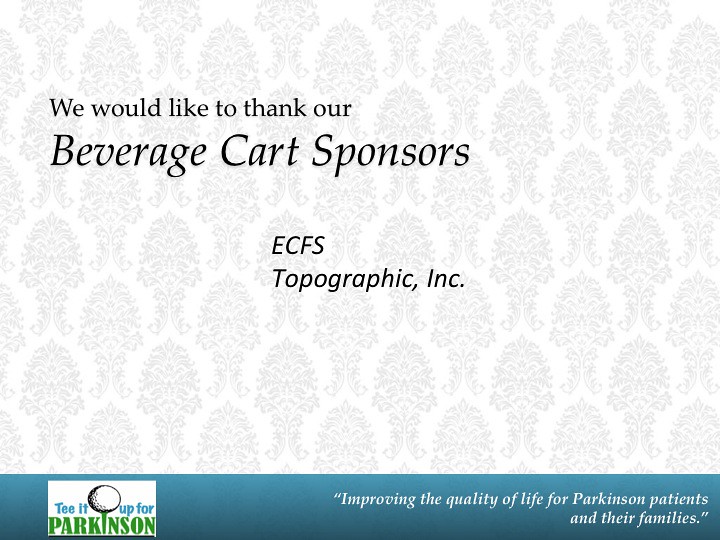The advertisement features a primarily white background adorned with a repetitive light gray floral pattern. Dominating the upper portion, approximately 80% of the image, is text in black lettering that reads, "We would like to thank our beverage cart sponsors, ECFS Topographic Inc." Below this, occupying the bottom 20% of the image, is a horizontal turquoise bar. On the left side of this bar is a logo consisting of a white box with a golf ball teed up, accompanied by the text "Tee it up for Parkinson's." To the right of the logo, in white letters, is the phrase, "Improving the quality of life for Parkinson's patients and their families." The overall design includes elements like trees sprouting with leaves forming a dome shape, adding an aesthetically pleasing touch to the visual presentation.